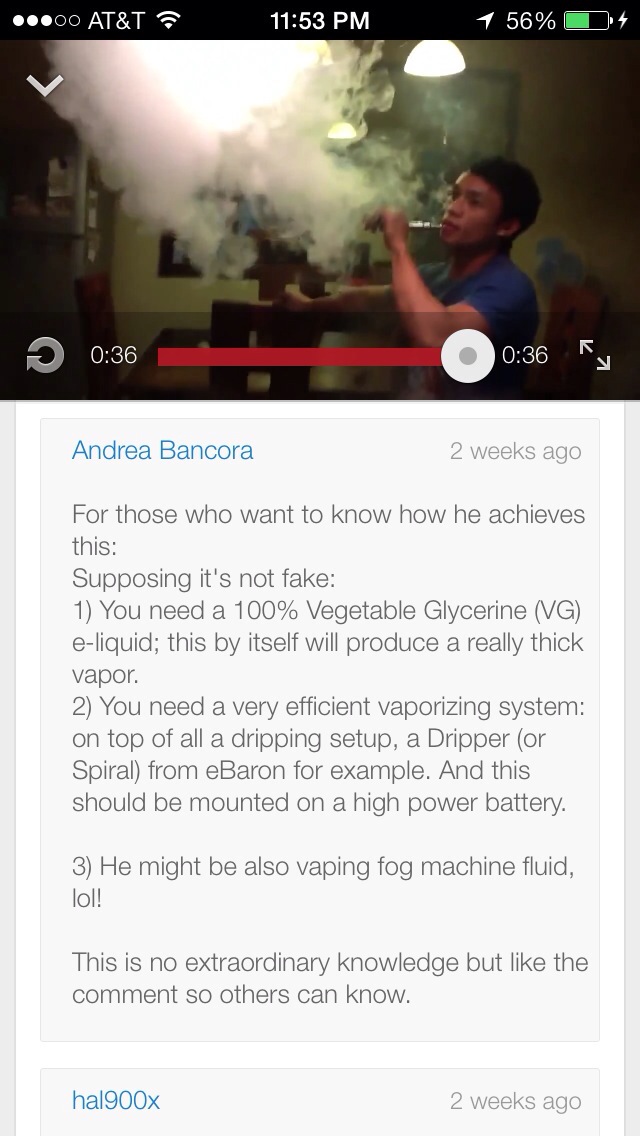The image is a screenshot taken from an iPhone, displaying a YouTube video and comments section. The status bar indicates the carrier is AT&T with the time at 11:53 p.m. and a battery level of 56%. In the video, a young man in a short-sleeved blue shirt is seen exhaling a large, billowy cloud of smoke, using a device that appears to be a vape or hookah. Below the video, a comment by Andrea Bancor, posted two weeks ago, explains the technique to achieve such thick vapor clouds. Andrea details that one would need 100% vegetable glycerin e-liquid, known for producing dense vapor, along with a very efficient vaporizing system, possibly recommending a dripper or spiral setup from eBaron, mounted on a high-power battery. They humorously suggest that the man might also be using fog machine fluid, and conclude by mentioning that this information is not extraordinary knowledge. The comment section ends with a prompt to like the comment so others can benefit from the information. The overall colors in the screenshot inclue gray, light blue, red, black, yellow, and green, typical of the YouTube interface on iOS.